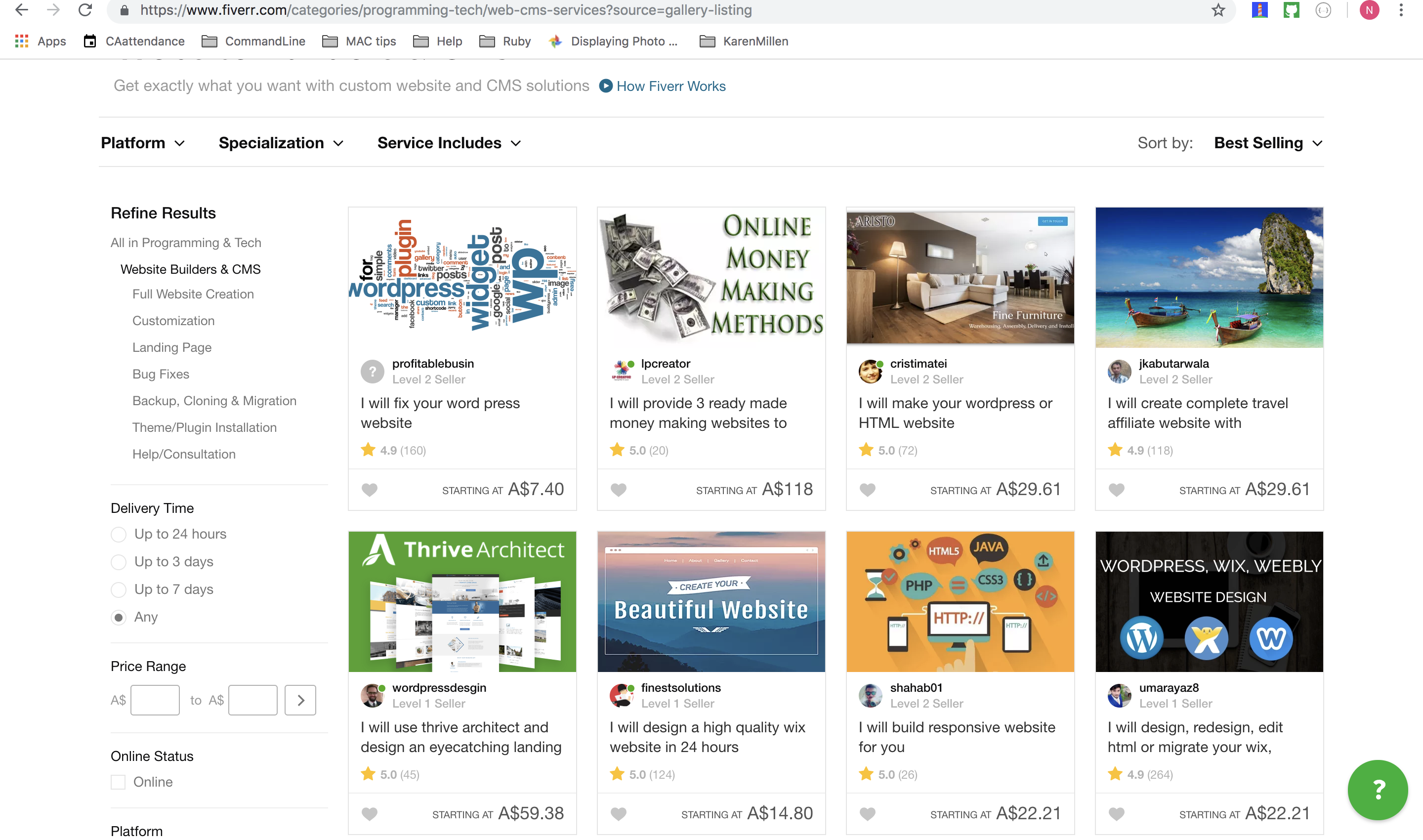The image showcases the Fiverr website, focused on offering custom website and CMS solutions. The URL displayed is "www.fiverr.com/category/programming-tech/web-CMS-services". The top of the page features a gallery of various services available for purchase, along with a prominent message that reads, "Get exactly what you want with custom website and CMS solutions." 

Below this message, there's a link titled "How Fiverr Works." The interface provides multiple filtering options like platforms, specializations, and service types, including categories such as "Full Website Creation," "Customization," "Landing Page," "Bug Fixes," "Backup, Cloning, and Migration," "Theme/Plug-in Installation," and "Help/Consultation." 

Users can also sort by "Best Selling" and refine results on the left sidebar, which offers additional filters for delivery time (up to 24 hours, up to 3 days, up to 7 days), pricing range, and online status. The selected category, "Website Builders and CMS," is highlighted and bolded.

The services listed include various offerings such as "I will fix your WordPress website," "I will provide three ready-made money-making websites," and "I will make your WordPress or HTML website," among others. Each listing promises expertise in website development and customization.